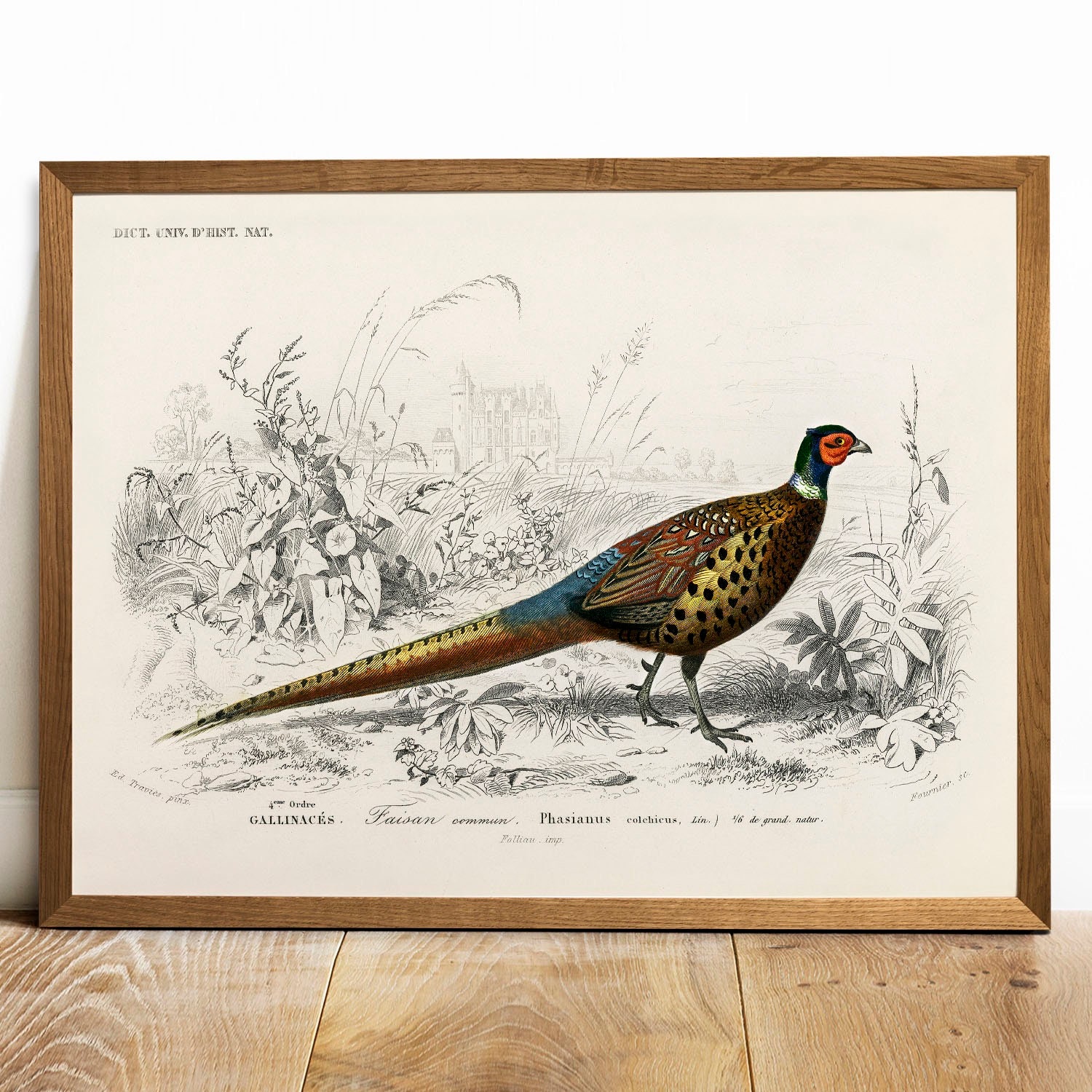This image shows a framed print of a colorful peacock, resting on a wooden floor against a white wall. The peacock, with its long tail not spread out, stands confidently facing right. Its plumage features a mix of browns, yellows, and beiges, while its head is black with a striking red face. The backdrop of the print is a black-and-white sketch, depicting an assortment of grass, leaves, and flowers, alongside some indistinct buildings, adding depth to the scene. At the top left corner of the print, the text "D-I-C-T-E-N-I-V" appears, and more text runs along the bottom, which is not in English and difficult to decipher. The blend of intricate details in the peacock and the monochrome background creates a striking contrast.